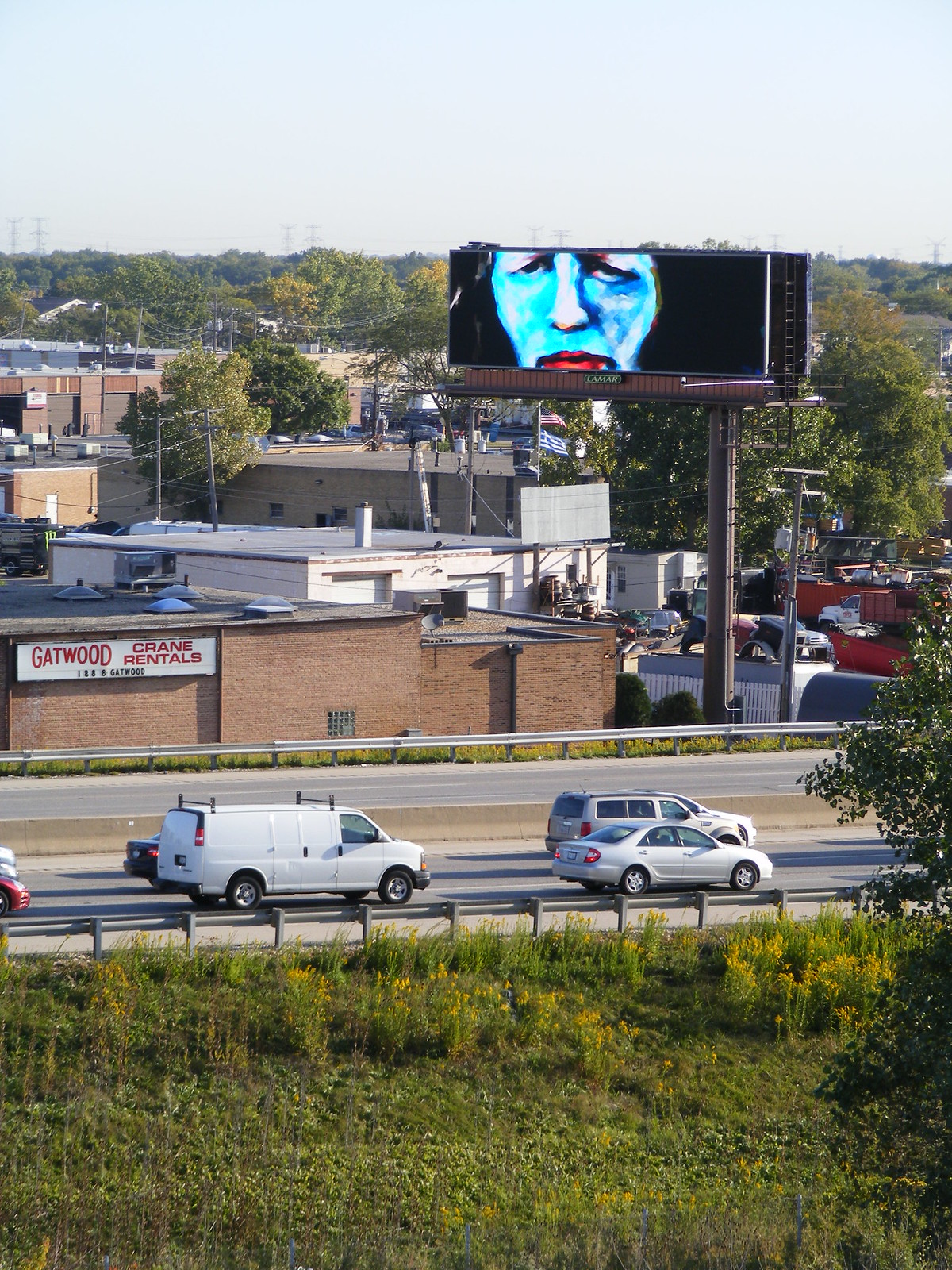An elevated vantage point offers a sweeping view of a green, grassy field descending towards the silver guardrails of a bustling highway. Taken perhaps from a hill or another high vantage point, this image has an older ambiance, suggesting it predates the common use of drones. The asphalt highway below is dotted with various vehicles, including a white van, an SUV, and several sedans, all contributing to the dynamic scene. Beyond the highway lies a row of short, flat-roofed buildings, one prominently displaying the sign "Gatwood Crane Rentals." The landscape is further characterized by scattered power lines and a cluster of trees. A striking feature in the background is a tall digital sign with a black background, displaying a noticeable frowny face, adding an intriguing element to the urban tableau.